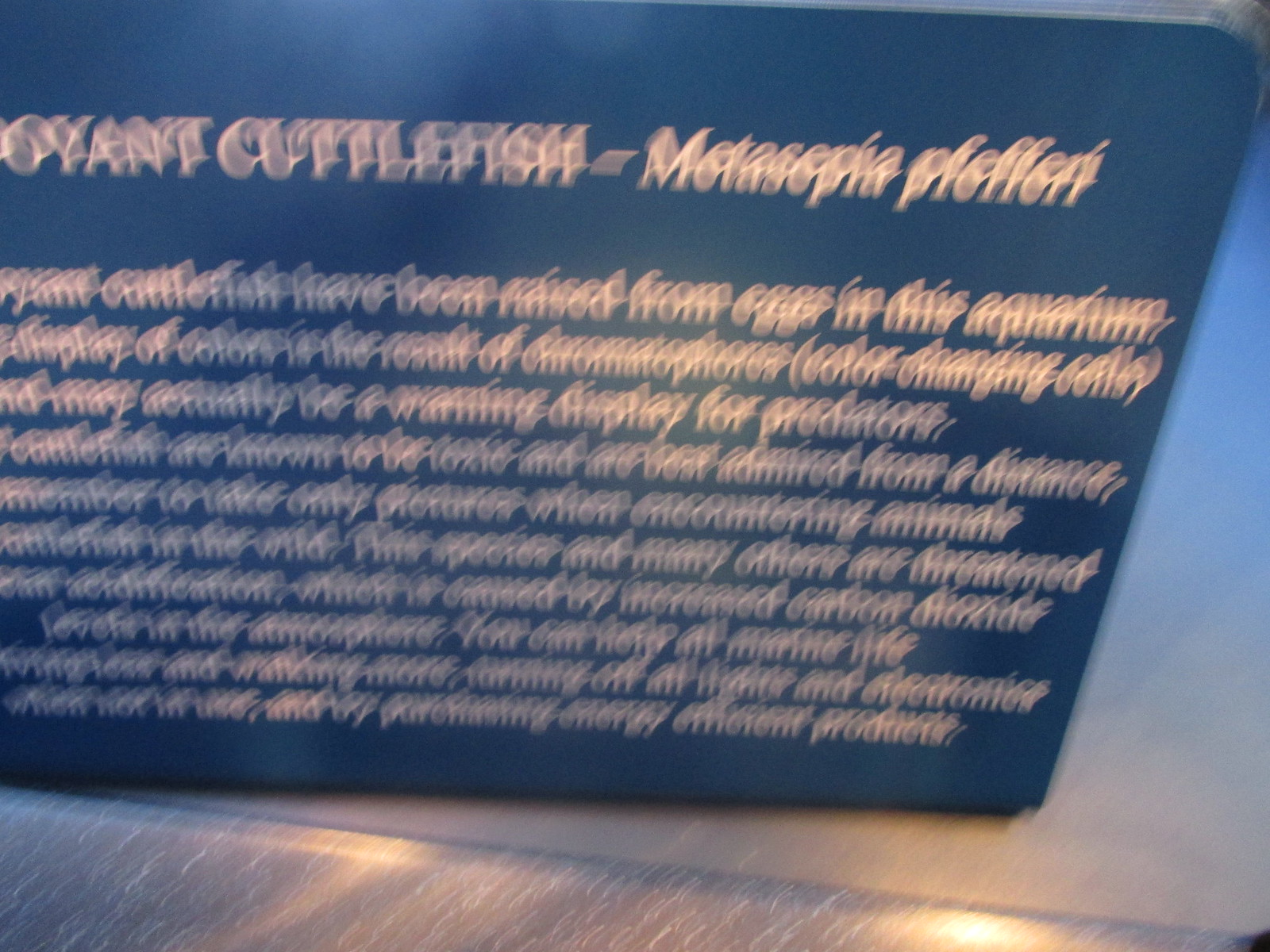The image shows a blue informational sign, likely located in an aquarium or marine-themed exhibit. The sign features white text, although the photograph is of poor quality, giving the image a double-vision effect that makes the writing difficult to discern. At the top of the sign, there's an identification of "cuttlefish," suggesting that this area of the exhibit focuses on these fascinating marine creatures. A paragraph of text below provides additional details, though it is largely unreadable due to the blurry and shaky nature of the photo. Key phrases such as "raised from eggs in this aquarium" are barely legible, hinting at the life cycle of the cuttlefish being highlighted.